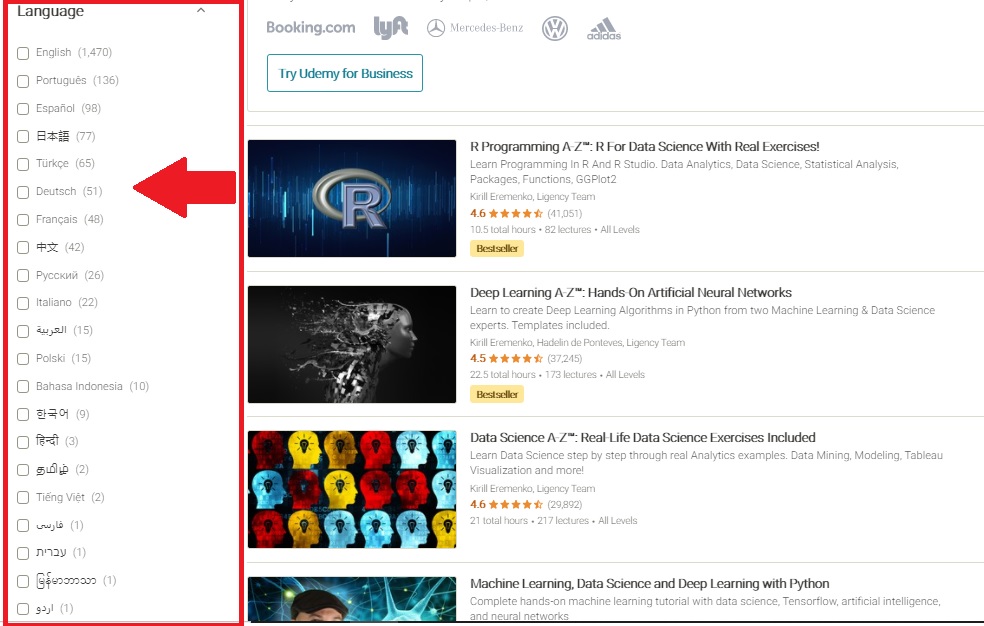The image depicts a complex webpage interface, likely a website for educational or business resources, heavily featuring familiar brand logos and language options. At the top, the logos of notable companies such as Booking.com, Lyft, Mercedes-Benz, Volkswagen, and Adidas are prominently displayed. On the right side, there's a vertical red-edged rectangle labeled "Language," containing a list of checkboxes for different languages. The first language listed is "English," with a count of 1,470 in parentheses. This is followed by languages like Portuguese and Español, as well as some Asian scripts that are not fully legible. 

Beneath the Booking.com logo, there is a rectangular box labeled "Try Udemy for Business," hinting at the educational focus of the site. Below this prompt, there are four images organized vertically, each representing different online courses. The first course is titled "R Programming A to Z," marked with an "R" icon. The second course is "Deep Learning," showcased with a computer-generated graphic. The third course, "Data Science A to Z," and the partially visible fourth course, "Machine Learning, Data Science, and Deep Learning with Python," follow suit. Notably, three of these courses have ratings, and two feature a "bestseller" badge, indicating their popularity.